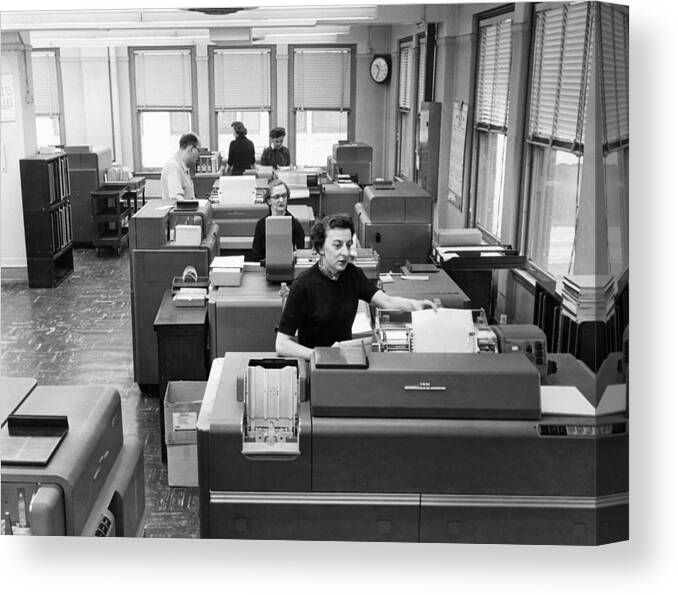This black-and-white photograph, likely from the 1950s, captures a bustling office scene featuring four women and one man engaged in their work. The office is spacious with several large windows on two walls, flooding the room with natural light. The floor is tiled in black with colored splashes, giving it a distinctive pattern.

In the foreground, an older Caucasian woman, dressed in a black dress with sleeves reaching her elbows, stands at a large copier, retrieving paper from the tray. Her black hair is neatly pulled up off her forehead. Behind her sits another older Caucasian woman, with tightly pinned-back hair, wearing glasses. She is engrossed in her work at a desk that houses a sizeable mechanical typewriter.

Further into the room, a Caucasian man with a balding head and glasses stands by another desk, possibly distributing documents. He is dressed in a short-sleeved, button-down collared shirt. Near the window at the back of the room, there are two more women. One woman is seated, typing with her head down, while the other stands with her back to the camera.

The walls are lined with various pieces of office equipment, including additional printers and typewriters. A clock in the back corner reads 10:35, keeping everyone on schedule. To the left, there are about five windows with shades partially drawn. The right side of the room features a bookcase halfway down, holding various documents and office supplies. The detailed setup and the busy atmosphere suggest a well-organized, mid-20th century office environment, where each individual is focused on their specific tasks amidst the era's characteristic furnishings and technology.